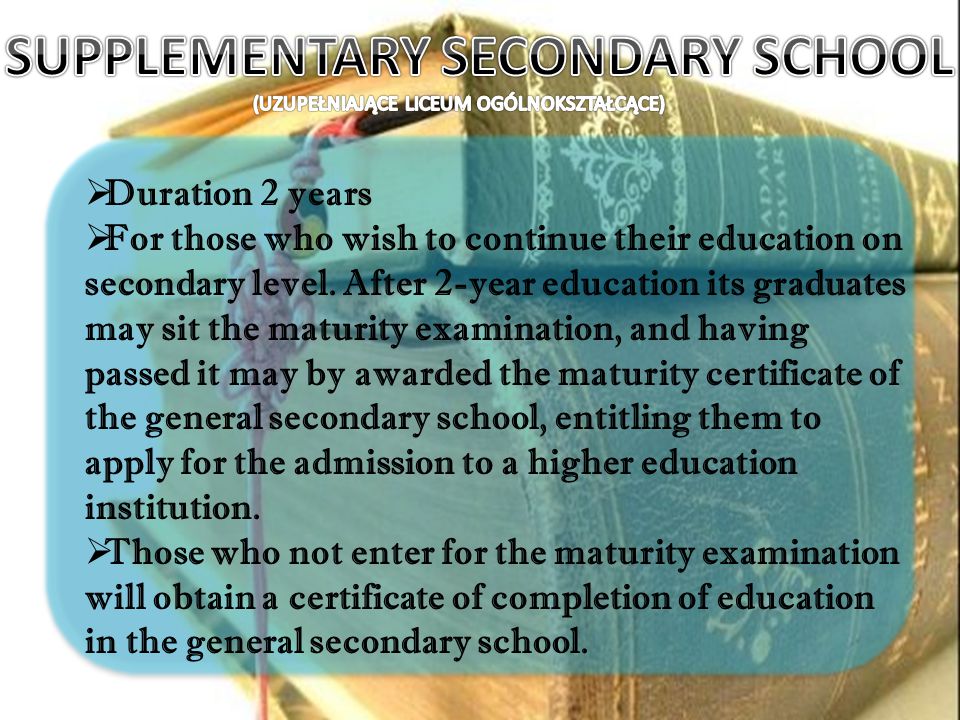This PowerPoint slide seems to be geared towards educational information about a supplementary secondary school. The background features a photograph of two stacked books, angled slightly, with old leather bindings. The books appear brown with gold leaf accents and ornate designs. The top book includes a visible bookmark cord with beads. The text on the slide is prominently superimposed over this backdrop. At the top, in bold black capital letters with a white outline, it reads "Supplementary Secondary School." Beneath that, in white text within brackets, is the phrase "Uzupeliniajas Lyceum Ogonokstalkasi." Following this, a large pale blue transparent box contains key details: 

1. "Duration: Two years."
2. A comprehensive description of the supplementary education, explaining that graduates may sit for the maturity examination to earn a maturity certificate, which qualifies them for higher education admission.
3. A note stating that those who do not take the maturity examination will receive a certificate of completion of education in the General Secondary School.

Overall, the detailed and ornate design of the slide, combined with the clear informative text, effectively communicates the supplementary educational pathways available.